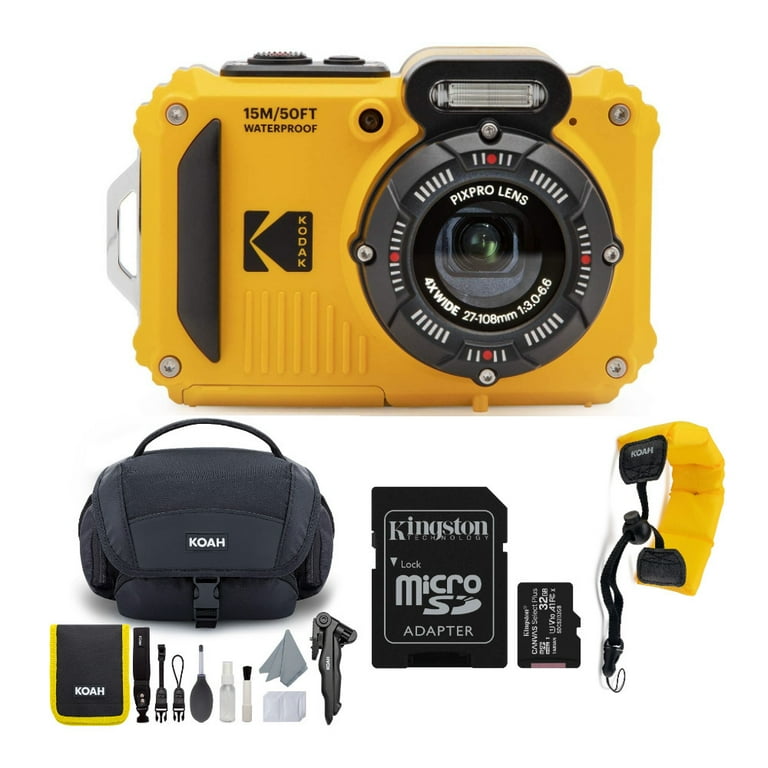This advertising image showcases a comprehensive underwater camera kit centered around a yellow, plastic-bodied Kodak waterproof camera. The camera, presented front-on, reveals its PixPro lens with specifications noted as 27-108mm, 4x wide. Prominent text on the camera body indicates its waterproof capabilities up to 15 meters or 50 feet. Additional details include a built-in flash, a silver bracket on the left side presumably for a strap, and a few buttons atop the camera.

Below the camera, a detailed assortment of accessories completes the kit. Dominantly featured is a black KOAH camera bag, accompanied by various maintenance tools including a lens cleaner, a multi-tool, brushes, a squeezable air blower, and a lens cloth. Central to the layout is a Kingston micro SD adapter with a small 32GB micro SD card positioned next to it. To the right of these items is a yellow KOAH strap, likely an inflatable safety mechanism designed to keep the camera afloat if dropped underwater.